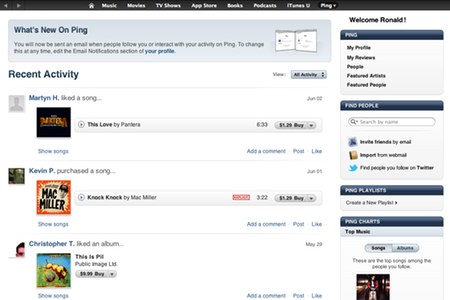The image depicts the interface of a music social platform called Ping, where users can share and discover favorite tracks and albums. At the top of the screen, a section titled "What's New on Ping" highlights recent activities within the community. On the left side, the latest interactions are showcased: one user has been listening to "This Love" by Pantera, another user purchased "Knock Knock" by Mac Miller, and a third user expressed approval for a recent album by Public Image Ltd., recognizable by its distinctive cover art.

On the right side, a personalized welcome message greets the logged-in user, whose name is Ronald. Under the "Ping" heading, Ronald can navigate through various sections of his profile including "My Reviews," "People," "Featured Artists," and "Featured Playlists." These sections emphasize the platform’s focus on user-generated reviews and community engagement.

A search bar is conveniently positioned beneath these options, allowing users to easily find music, reviews, and other content on the site. The overall layout and features affirm that Ping is designed to facilitate music discovery, reviews, and social interaction among its users.